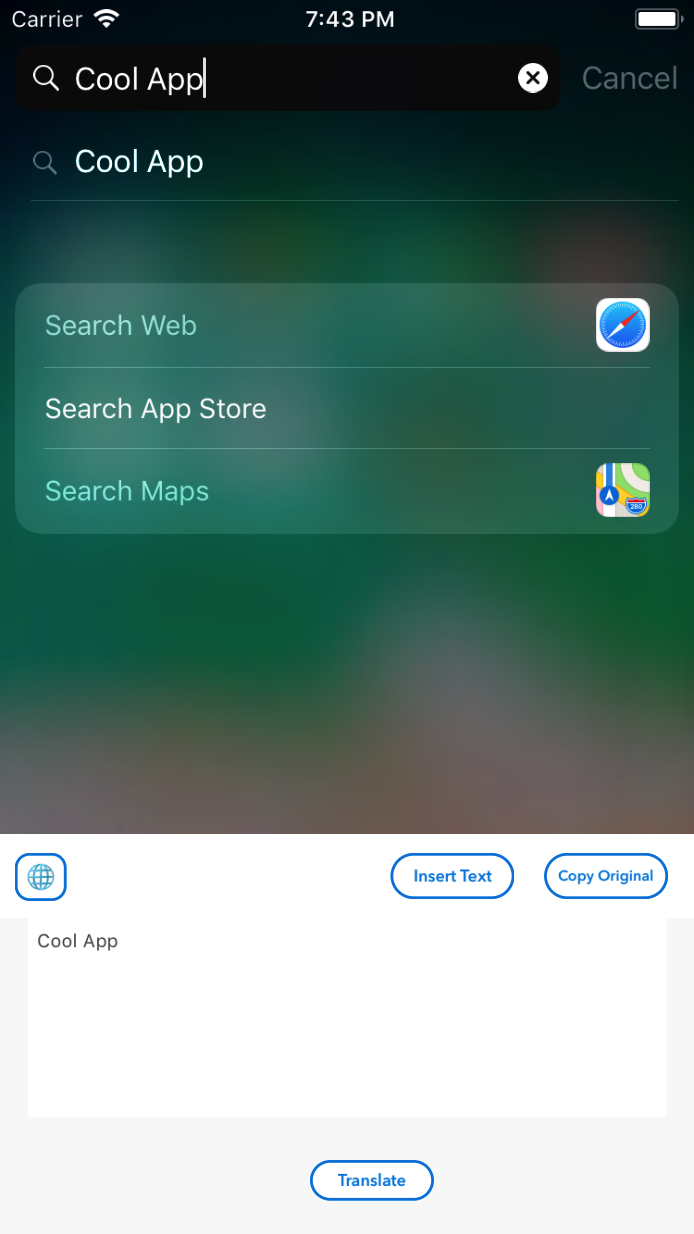A screenshot displays a smartphone interface with a gradient-colored background that transitions from charcoal gray at the top, to light gray, then dark green, and eventually a grayish-pink hue at the bottom. 

At the top left corner, "Carrier" is displayed alongside a Wi-Fi signal icon, while the center shows "7:43 p.m." The far right reveals a battery icon indicating a full charge. Below the time, a text box with the label "Cool App" appears, featuring a search glass icon on the left and a white circle with an "X" on the right, accompanied by the word "Cancel."

Beneath this, the text "Cool App" reappears, indicating a previous search. Centrally located on the screen is a light green rectangular button labeled "Search Web," next to which is a small icon. Directly beneath, "Search App Store" and "Search Maps" are listed, each with their respective Google icons.

At the bottom of the screen, there is a gray bar containing a globe icon, flanked to the right by two elongated oval buttons labeled "Insert Text" and "Copy Original." At the very bottom, an oval button labeled "Translate" completes the interface.